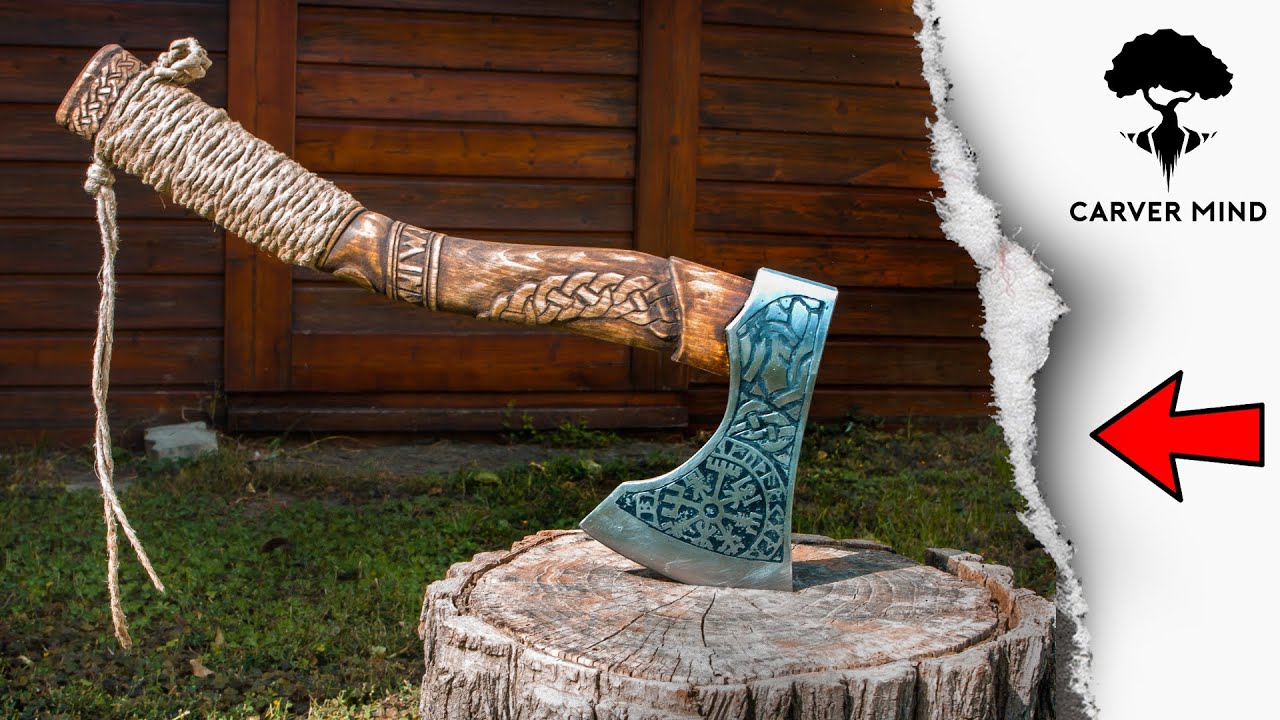This image showcases a highly ornate hatchet embedded into an old tree stump, which sits on a patch of short grass with a dark wooden fence in the background. The handle of the hatchet is wooden and intricately carved, featuring a braided pattern running down the shaft and additional carvings at the bottom. A segment of the handle is wrapped with rope or twine, which is tied into a knot with two ends hanging loose. The hatchet's blade is made of bluish silver metal, engraved with detailed decorations, including a circular design on the front and Viking-like symbols towards the back.

On the right side of the image, the background turns white, containing a black silhouette of a tree on a floating cliff with the text "Carver Mind" beneath it. Just below this, a red arrow outlined in black points towards the hatchet embedded in the tree stump.